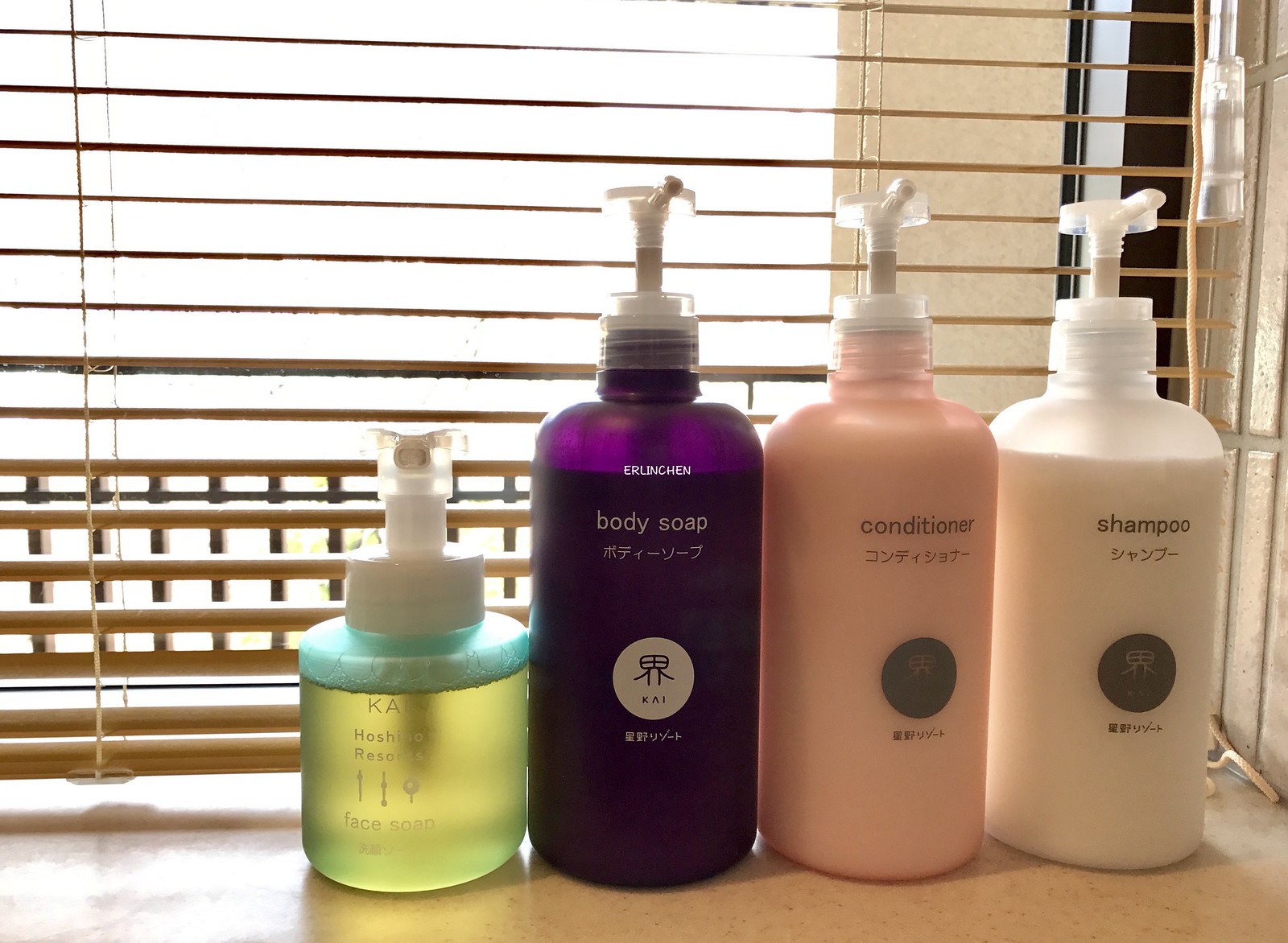A well-organized lineup of four personal hygiene products is showcased against a softly lit backdrop. 

Starting from the left, there's a small, cylindrical perfume bottle with a slightly opaque, pale yellow liquid inside, visible bubbles, and a label that reads "K". This bottle features a white lid extending into a white spray nozzle with an accompanying plastic cover.

Next to it is a taller, cylindrical purple bottle with subtly rounded corners. This container is labeled "Girl Legend Body Soap" in English and East Asian text. The bottle has a translucent plastic pump at the top, revealing its functionality. 

To the right of the body soap bottle are two similar-shaped containers, distinguished by their colors and labels. The middle one, a pink bottle marked "Conditioner", sports a light gray emblem in the center. Finally, the white bottle labeled "Shampoo" is slightly used, showing some product at the top, and has the same light gray emblem in the middle as the conditioner.

The background features a window with open blinds, allowing natural light to softly illuminate the scene. To the top right, a tan building can be seen through the blinds, along with a black fence or gate that doesn't obscure the view. The plastic handle and string of the blinds are also visible, indicating a bright and clear day outside.